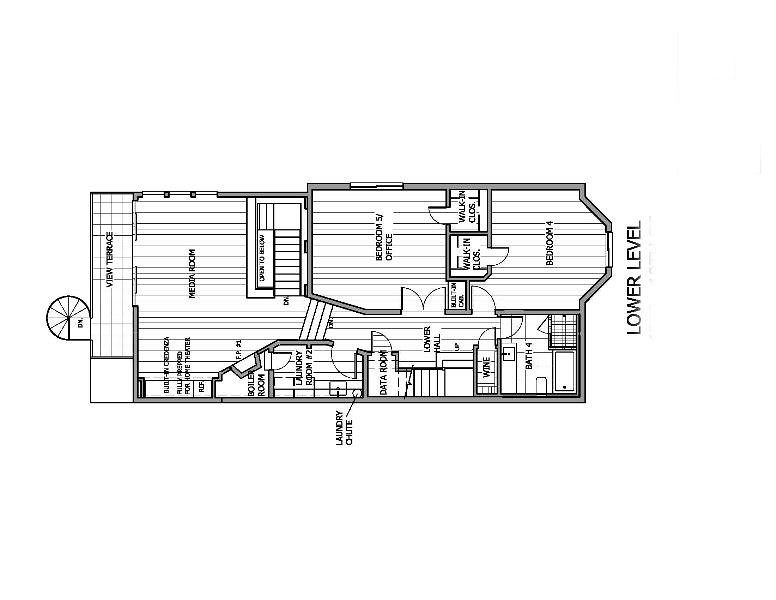This detailed blueprint image, illustrated in black and white, appears to have been meticulously drafted, likely using computer software. Displayed sideways, the blueprint represents the lower level of a multi-story building. Key features include numbered rooms such as a bathroom, a dedicated wine room, bedroom four, and bedroom five, which is designated as an office. The blueprint also outlines functional spaces including walk-in closets, a laundry room complete with a laundry chute, and a boiler room. Additionally, it marks a media room and another, less legible room near a view terrace. A unique feature depicted is an area referred to as "open to below," suggesting a mezzanine or open space adjacent to a staircase. Interestingly, a Ferris wheel is sketched on the far end of the layout, adding a whimsical element to the design. The blueprint focuses solely on the lower level, with no depiction of the upper levels at this time.